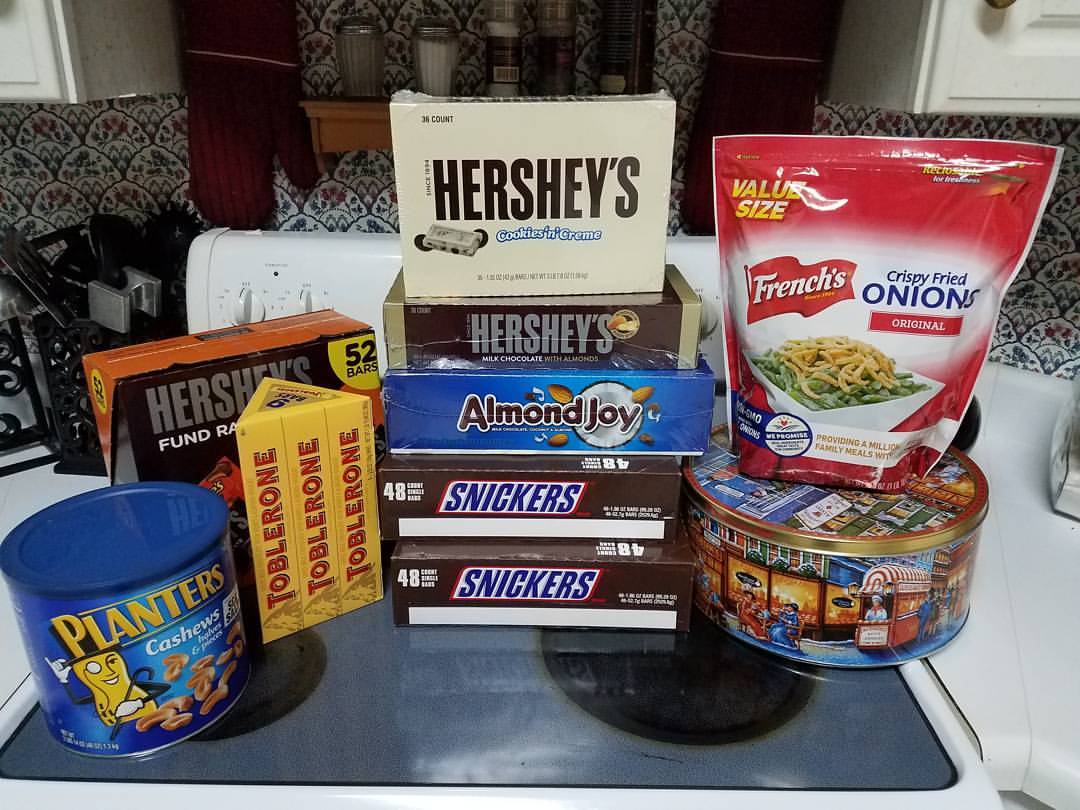The image features an assortment of candy and snack boxes arranged on a grey stovetop with black electric burners, surrounded by a white countertop. Prominently featured in the center are two rectangular Snickers boxes in brown, adorned with the iconic blue Snickers logo and the number "48" in blue text at the bottom. Above the Snickers boxes is a rectangular Almond Joy box in blue, topped with a brown Hershey's box, and finally, a Hershey's Cookies and Cream box sits at the very top.

To the right of this central stack, there is a circular tin holding a red and white plastic bag of French's crispy fried onions. On the left side of the central chocolate boxes are multiple Toblerone boxes, a Hershey's Fundraiser rectangular box, and a blue cylindrical tin can of Planters Cashews. The overall arrangement showcases an enticing variety of sweets and snacks.